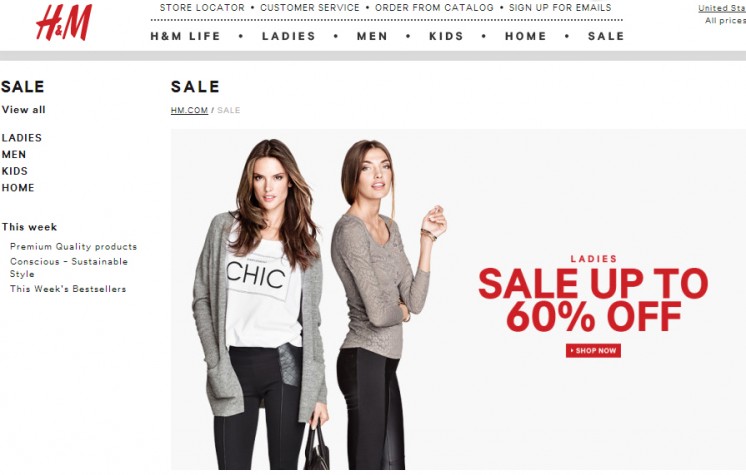This is a cropped screenshot of the H&M website with a white background. At the top left corner, the iconic H&M logo is displayed in red. Moving to the right, centrally aligned at the top, are navigational links: "Store Locator," "Customer Service," "Order from Catalog," and "Sign Up for Emails." Below this navigation menu, another row features sections such as "H&M Life," "Ladies," "Men," "Kids," "Home," and "Sale."

A thick gray horizontal line extends across the width of the page, creating a separation between the header and the main content. On the left side of the page, the word "Sale" is prominently displayed in bold black letters at the top. Below this, options are listed including "View All," followed by subcategories "Ladies," "Men," "Kids," and "Home." Further down, in smaller black text, it reads "This Week," under which categories like "Premium Quality Products," "Conscious," "Sustainable Style," and "This Week's Best Sellers" are mentioned.

On the right side, at the top, "Sale" is also highlighted in bold black letters. Directly beneath it, the URL "HM.com/sale" is shown. Dominating the center of the page is a large square photo featuring two models showcasing H&M clothing. Adjacent to this image, a promotional banner states "Ladies, Sale up to 60% off, Shop Now." The remainder of the website is not visible in this cropped view.